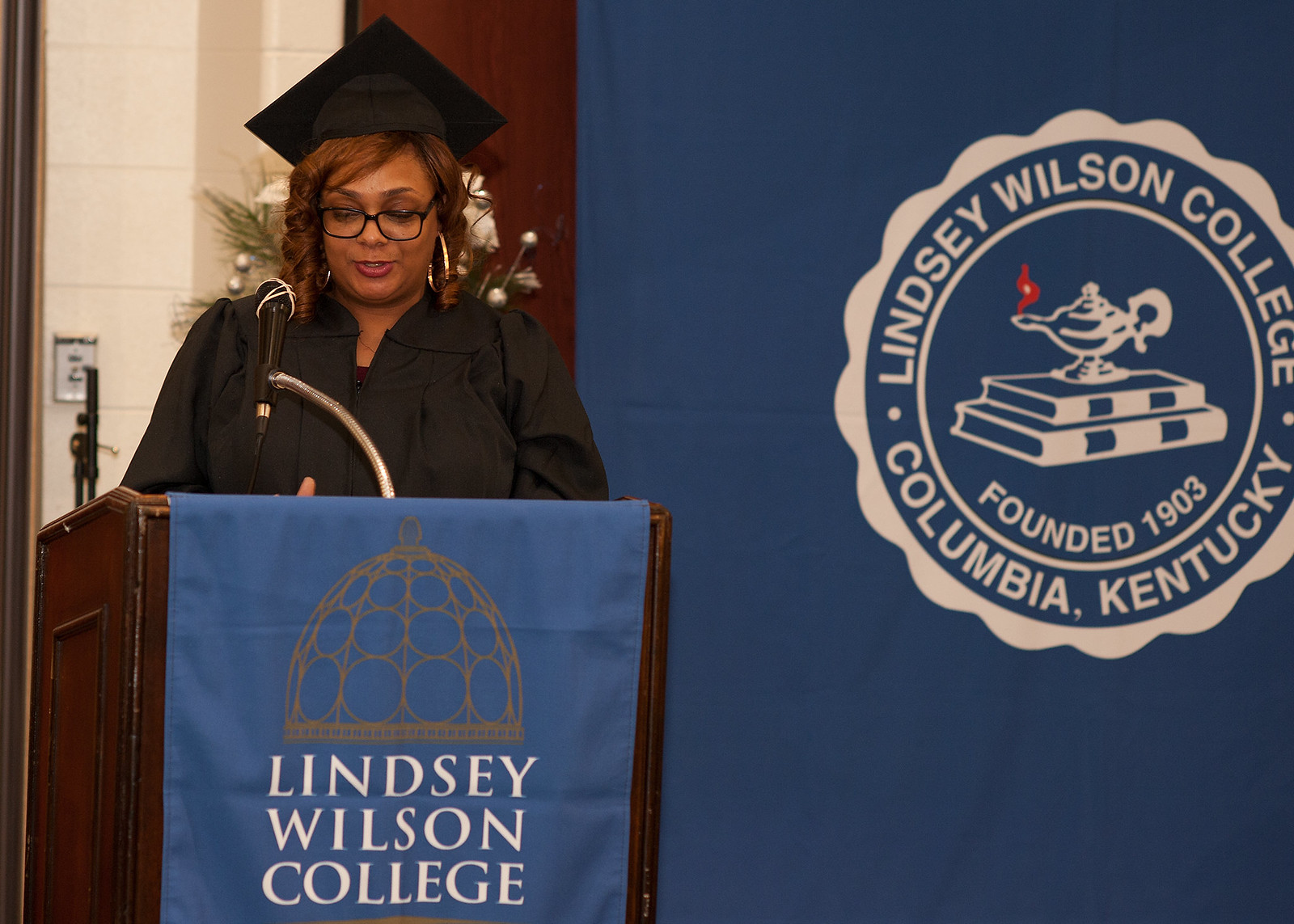The photograph captures an indoor college event, prominently featuring a woman standing to the left side behind a wooden podium. She is a young black woman adorned in a black graduation gown and cap, with her dark brown, curly hair falling to her shoulders. She accessorizes with large golden hoop earrings and black-rimmed glasses, complementing her light red lipstick. The woman appears to be reading from a sheet of paper placed on the podium, with a microphone positioned in front of her, noticeably secured with rubber bands around its top. 

The podium bears a cloth banner with "Lindsay Wilson College" emblazoned in white lettering. Behind her, the setting is characterized by a brick wall and another larger, blue banner hanging to the right. This banner features a circular seal stating "Lindsay Wilson College, Columbia, Kentucky" around the perimeter, with "Founded 1903" underneath. At the center of the seal, there is an illustration of a magical lamp emitting red smoke, positioned atop two stacked books.